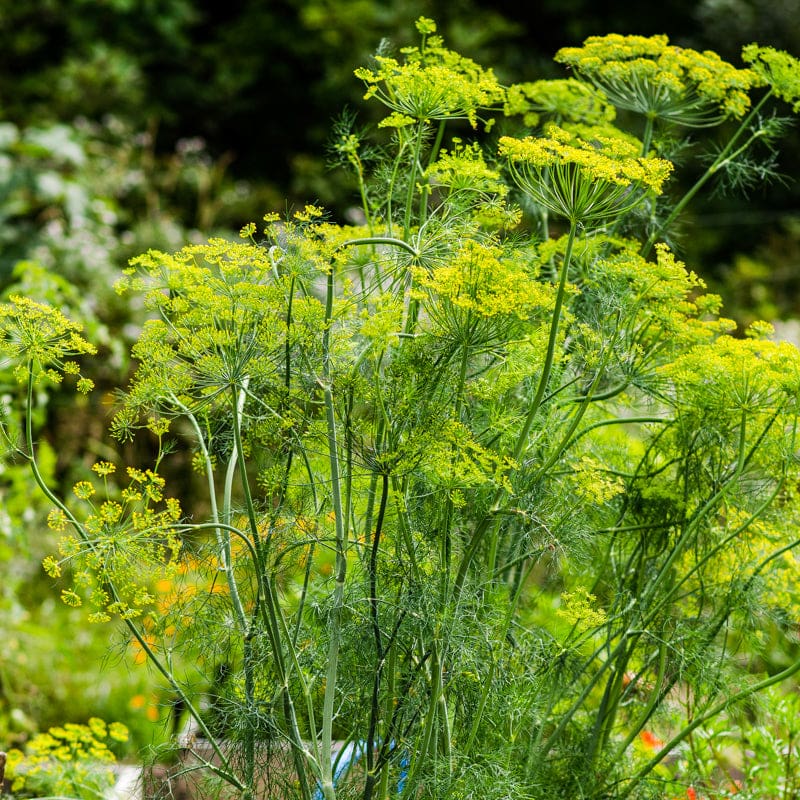In this detailed photograph taken outdoors, the focal point is a cluster of wild carrot flowers thriving in a grassy field. These plants, marked by their slender, long dark green stems, stand about two and a half to three feet tall. The flower heads bloom in intricate clusters, each larger flower composed of many tiny flowers nestled together. Predominantly green and yellow hues dominate the scene. The flowers feature small green centers with delicate yellow dots encircling them, contributing to the vibrant coloration. Toward the upper right-hand corner, there are wispy white hairs that resemble cotton or webbing clinging to the plant. In the background, less detailed white flowers can be seen. The image also hints at a brown outline at the bottom, suggesting the plants may be rooted in flowerbeds. Notably, wild carrot plants have medicinal uses but can also pose a danger if ingested or touched by those sensitive, as contact dermatitis may occur.